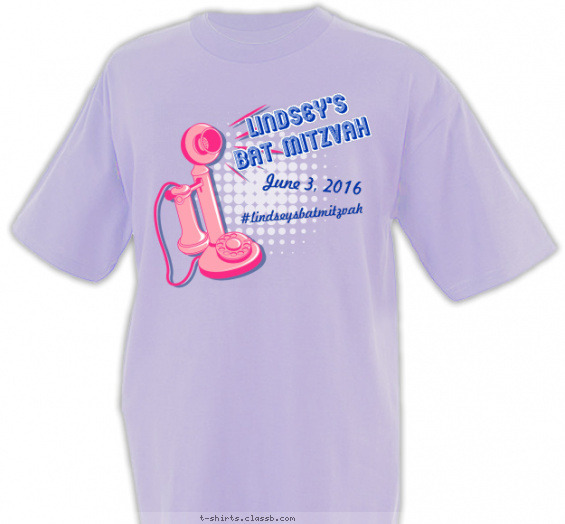This image depicts a light purplish lavender commemorative t-shirt with short sleeves. Positioned centrally on the chest, the design features a vintage 19th-century style telephone in various shades of pink, resembling an antique rotary phone. This phone is set against a white disco ball background that adds a striking contrast. Adjacent to this retro phone, in bold blue lettering encased in a subtle white outline, the t-shirt reads "Lindsay's Bat Mitzvah, June 3rd, 2016," with the phrase "#LindsaysBatMitzvah" directly beneath it. The text is both prominent and eye-catching, with the date and hashtag subtly italicized for emphasis. At the bottom of the image, separate from the t-shirt design itself, is the website t-shirts.classb.com, suggesting that this photo serves as an advertisement for custom t-shirts available from that particular site.